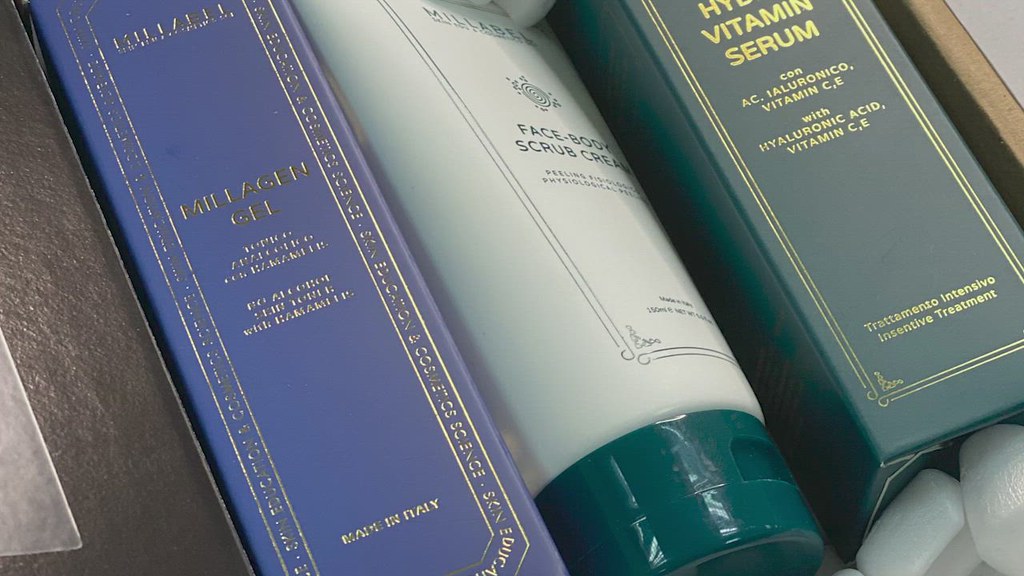The image is an up-close shot of an unboxing of skincare products, focusing on three distinct items nestled within a grey cardboard box. The scene reveals white packing peanuts in the lower right corner and a few scattered at the top center. The first item is packaged in an elegant blue box adorned with gold writing, which appears narrow and somewhat difficult to decipher. The legible text suggests it may say "Milligan," along with "Made in Italy." 

The second item is a white tube capped with green, clearly labeled as "Millibel Face Body Scrub Cream." 

The third item is a green box with gold lettering and trim. While the top part of the text is obscured, partially visible letters "H-Y" can be seen. The box prominently displays "Vitamin Serum" and further clarifies its contents with the text "Con A.C. Hyaluronic Vitamin C, E With Hyaluronic Acid Vitamin C and E." At the bottom, it is labeled "Tratamento Intensivo," translating to "Incentive Treatment."